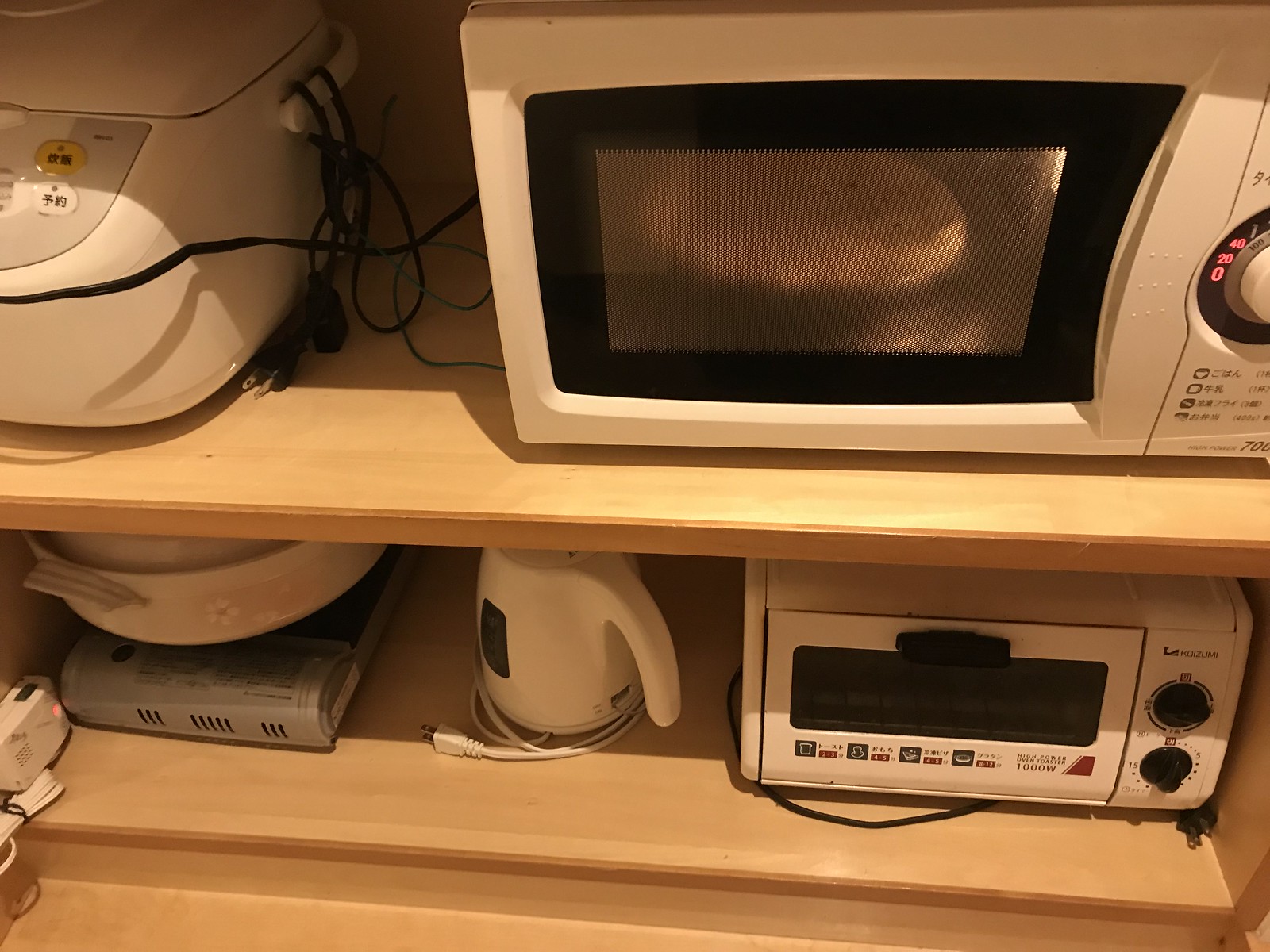This color photograph showcases a wooden cabinet with two shelves, heavily lined with various small kitchen appliances. Dominating the top right corner is an active, white microwave oven with a black-framed glass door, through which a pot pie or similar item is visible, illuminated by the microwave’s internal light. The microwave dial prominently displays numbers, including 40, 20, and 0. To the left of the microwave, there is what appears to be the base of a blender adorned with foreign lettering. Adjacent to it, still on the top shelf, is a white rice cooker with multiple plugs trailing behind it.

On the bottom shelf, starting from the left, there's a small gas plate covered by a white bowl adorned with floral patterns, positioned atop a gray scale. Moving right, a white electric kettle rests beside a white extension cord. Further right sits a white toaster oven, unplugged, with black handles. All these appliances are meticulously placed on light wooden shelves, embodying a compact yet organized kitchen storage setup.